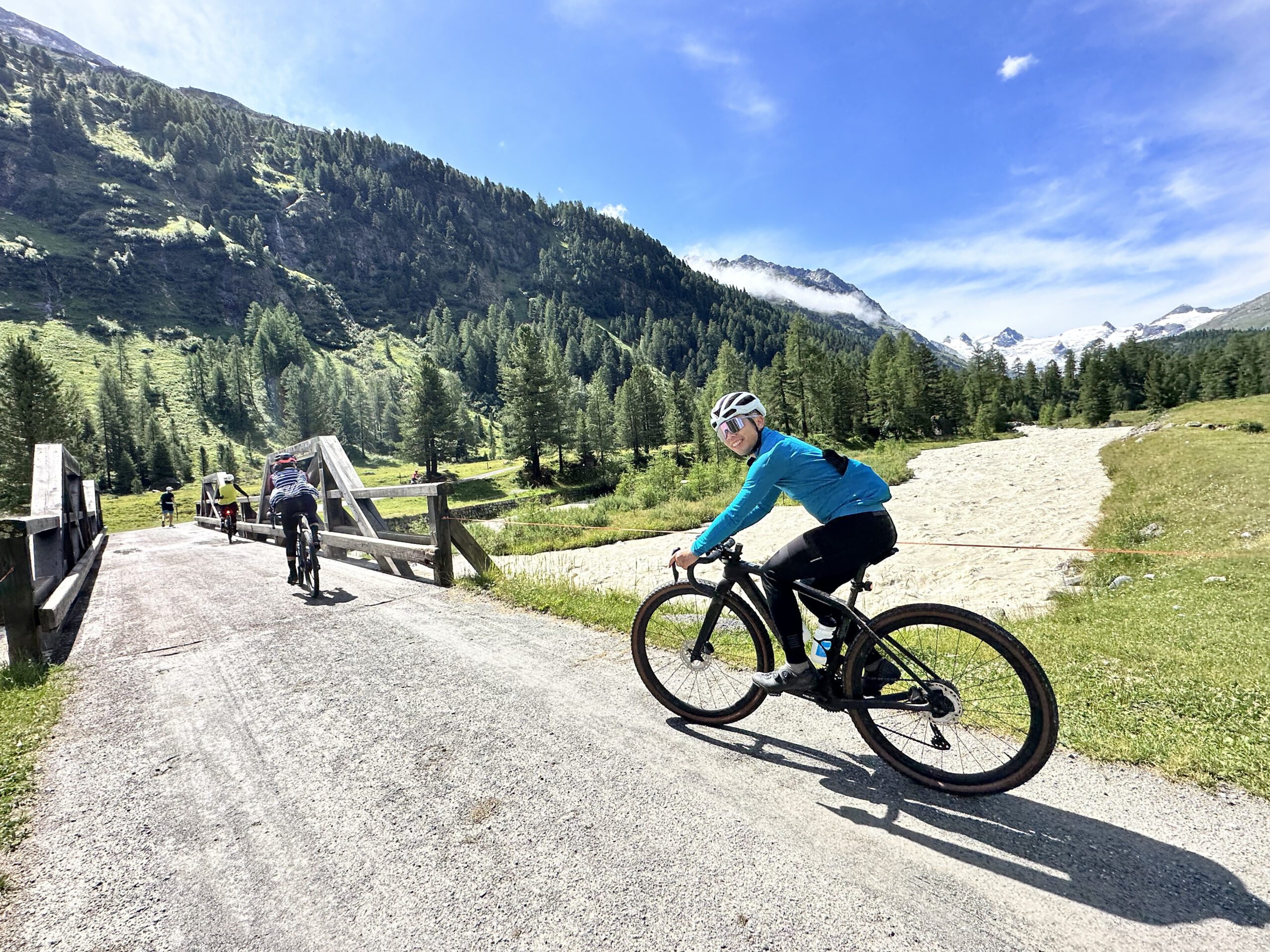This detailed outdoor daytime photograph features a white, male cyclist in the foreground, prominently positioned from the bottom left corner to the center. The cyclist is riding a black mountain bike without fenders, wearing black pants, a light blue long-sleeve shirt, a white helmet, and white sunglasses. He has a cheerful expression, turning his head to smile directly at the camera. 

In the image's background, three more cyclists are visible, aligned one after another, moving towards a wooden bridge. These cyclists have their backs to the camera as they cross the gravel path leading to the bridge. The scenic backdrop displays an expansive landscape where tall, green pine trees merge into lush grassy areas. Beyond the trees, large mountain ranges dominate the view, with the left side showcasing dark green, tree-covered hills and the right side revealing imposing gray mountains capped with snow. The sky above is a clear blue with scattered thin white clouds, adding to the picturesque setting of this state park or nature reserve.